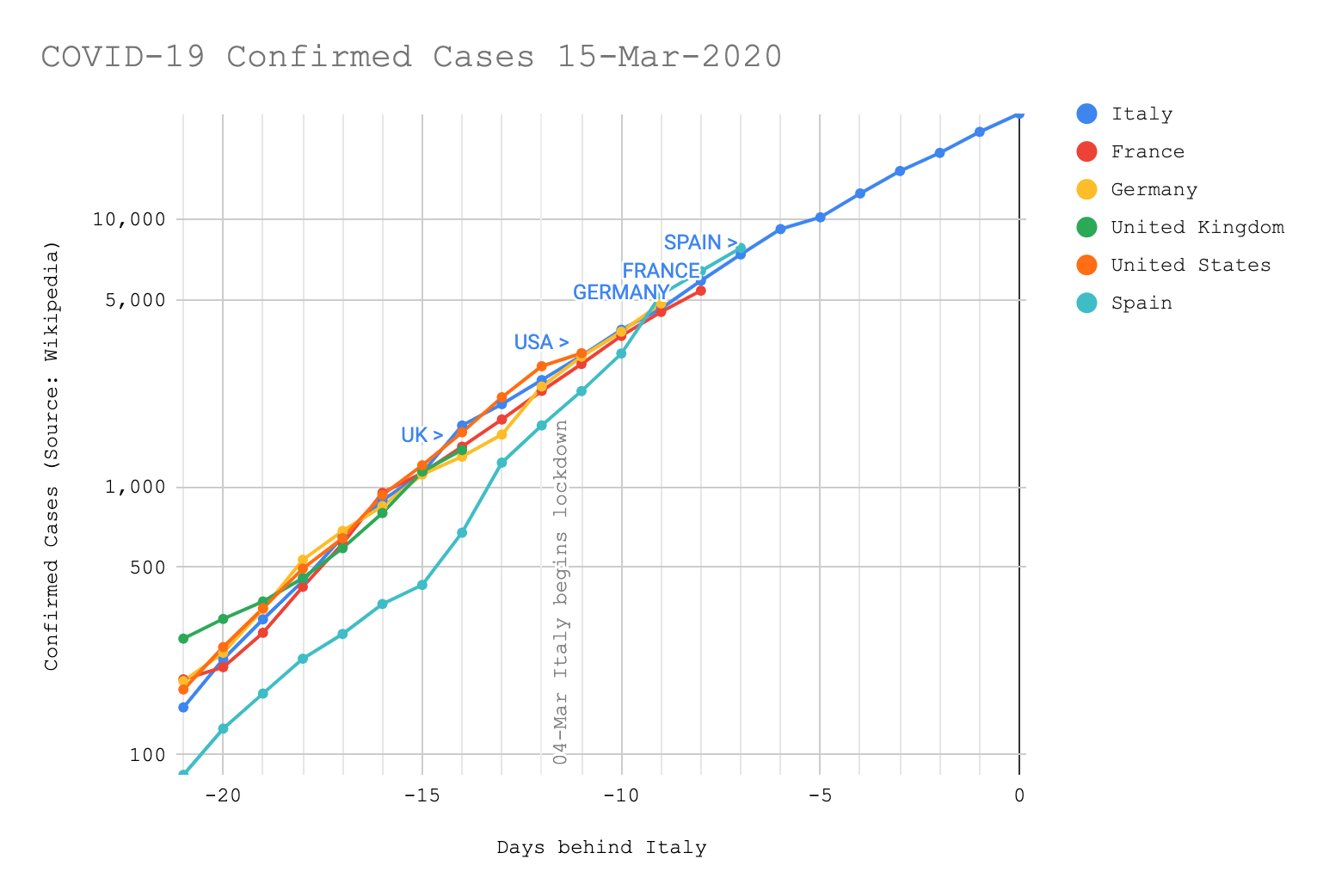The image depicts a graph illustrating the confirmed COVID-19 cases as of March 15, 2020, for six countries: Italy, Spain, France, Germany, the United States, and the United Kingdom. The x-axis represents the number of days past the first reported case, highlighting a comparative timeline among the countries, with Italy serving as the reference point. 

The y-axis enumerates the confirmed cases in increments of 100, 500, 1,000, 5,000, and 10,000, offering a clear view of the pandemic's progression in each country. Notably, Italy appears at the top with the highest number of cases, followed closely by Spain. France and Germany show a similar trend, trailing behind Spain. The United States follows next, with the United Kingdom recording the fewest cases among the listed countries. The source of the data is Wikipedia, as indicated in parentheses.

The visualization showcases the stark contrast between the rapid case acceleration in Italy compared to the slower increase in the UK, emphasizing the varying rates of COVID-19 spread across these nations.